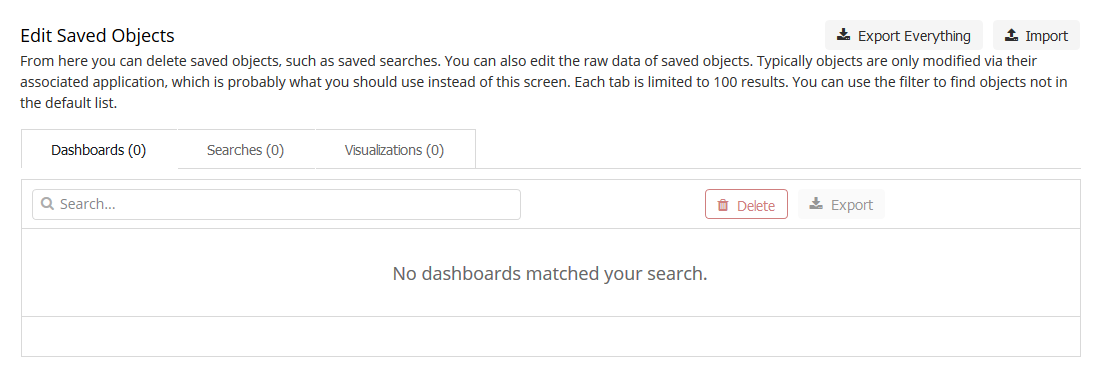This image is a screenshot capturing the "Edit Saved Objects" webpage of a website, dedicated to managing stored objects. The webpage features a clean white background with predominantly black text. 

At the top left corner, large black text displays the page title, "Edit Saved Objects." On the top right, there are two light gray buttons with black text: "Export Everything" and "Import," providing options for exporting or importing objects to the website.

Beneath the title, a paragraph of smaller black text outlines the page’s functionality: users can delete saved objects like searches, edit raw data of saved objects, and are advised that objects are typically modified via their associated application, rather than through this screen. It also mentions that each tab is limited to 100 results and advises using the filter to find non-listed objects.

Below this informational paragraph, there are three tabs labeled "Dashboards," "Searches," and "Visualizations." Currently, the "Dashboards" tab, indicated in black text, is selected, while "Searches" and "Visualizations" remain in gray text. 

Following the tabs, a search interface appears specific to the Dashboard objects. It features a red "Delete" button and another button labeled "Export." In the center of this section, a message states, "No Dashboards match your search," indicating that the Dashboard is empty and objects need to be imported to populate it.